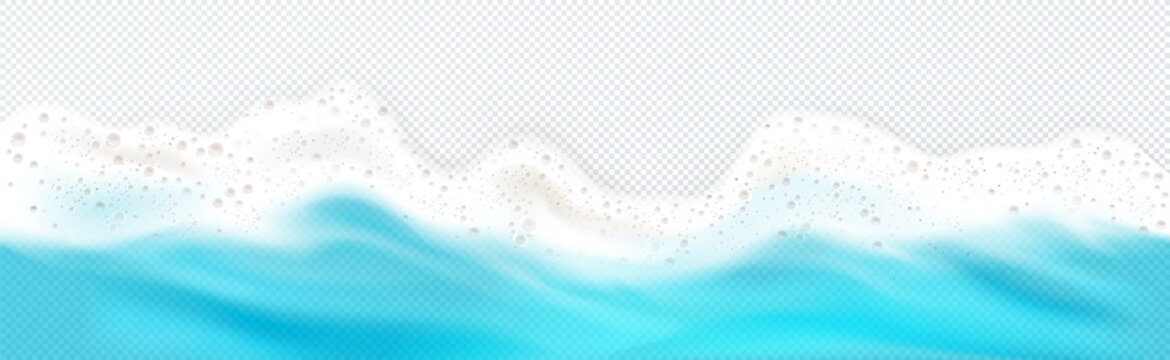The image depicts a stylized, computer-generated ocean view, characterized by its light blue, aquamarine waters with deeper blue shades providing a sense of depth and movement. The waves exhibit a frothy white foam at their crests, interspersed with gray bubbles of various sizes, giving an impression of dynamic sea foam. The background features a pixelated gray and white checkerboard pattern, formed by overlapping diagonal lines, reinforcing the transparency of the image. This rectangular image combines elements of light and dark blue shading to create a somewhat three-dimensional and animated effect, highlighted by the foamy white tips and the intricate checkerboard pattern suggesting the absence of further background detail.